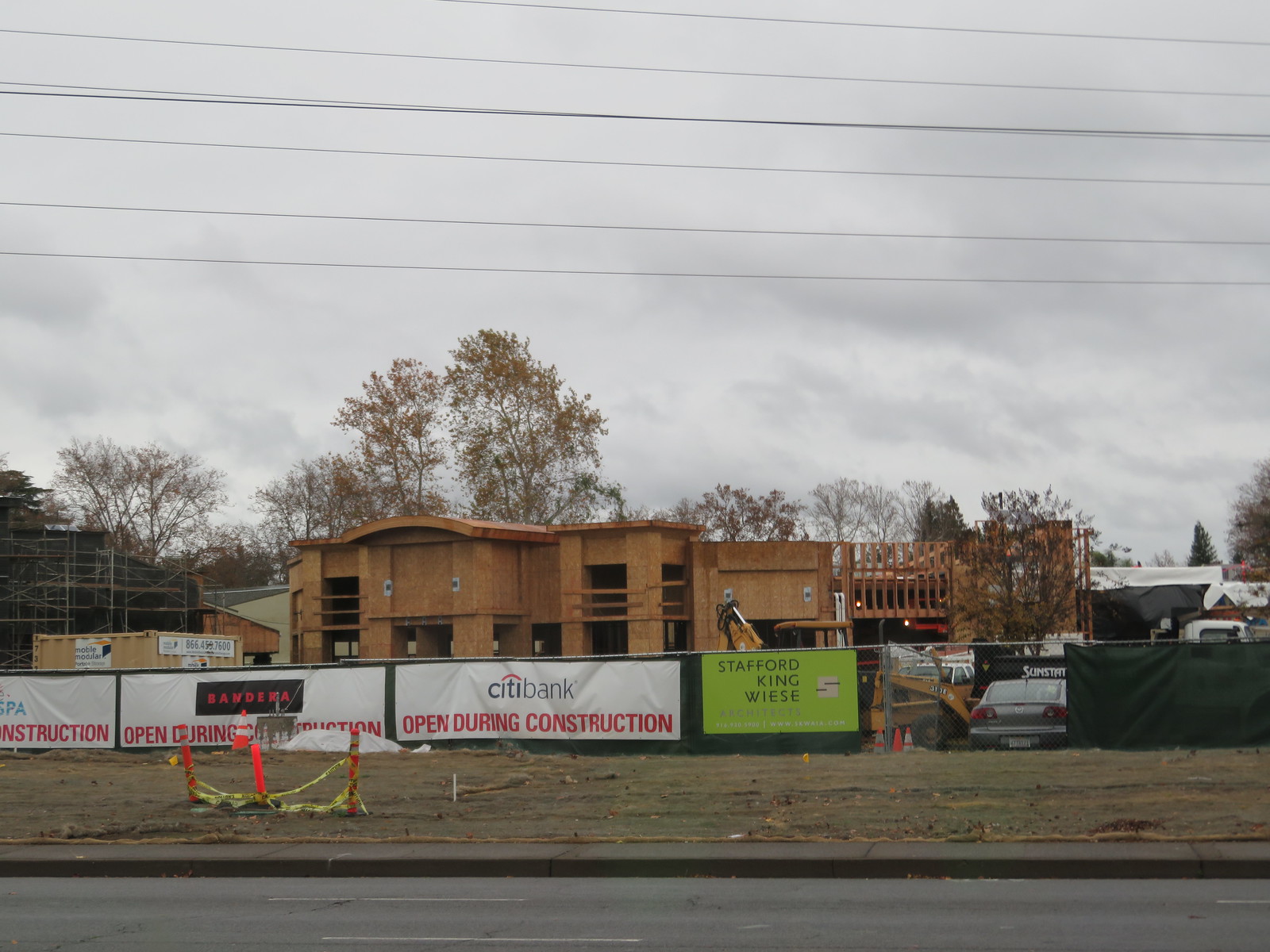In this image, a photograph captures a construction site situated across the street. The focus is on the wooden framework of a building under construction, devoid of its outer exterior. It prominently displays the future locations for windows and doorways. Surrounding the site is a silver chain-link fence adorned with multiple banners, including a white and red sign stating "Citibank open during construction" and another indicating "Stafford King Weiss Architects." Additional signage mentions "Bandera, open during construction."

In the foreground, the asphalt road transitions into a cement sidewalk, leading up to a patch of torn-up, lifeless grass encircled by warning tape. Various pieces of construction equipment and parked cars are visible within the site, enhancing the sense of ongoing development.

Trees displaying autumnal hues of orange and brown are scattered in the background, against a dark, overcast sky that suggests an imminent rain. The overall ambiance of the scene is one of bustling activity despite the dreary weather conditions.